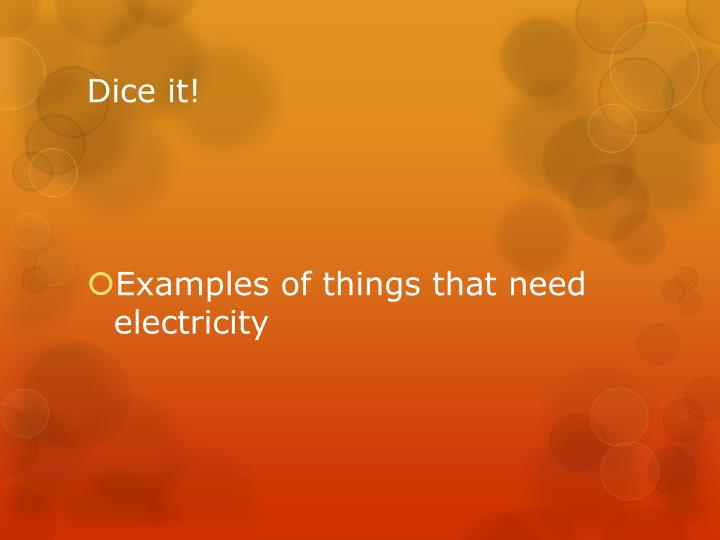The slide from our presentation features a dynamic orange and red gradient background, with orange at the top and red at the bottom. The corners of the slide are adorned with clusters of darker shaded circles, providing a subtle, textured contrast to the gradient. The slide's title, "Dice It!" is prominently displayed in white Arial font at the upper-left corner, emphasizing the theme energetically with an exclamation mark. Below the title, a single bullet point in white text, outlined with a yellow unfilled circle, reads "Examples of things that need electricity." This minimalist yet vibrant design draws attention to the key elements of the presentation.